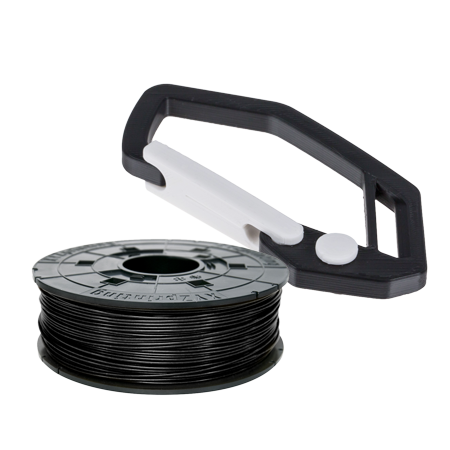In this image, we observe a collection of hardware items set against a neutral background. To the left, there is a black, relatively flat plastic spool. Wrapped intricately around this spool is a thin, black material that appears to be either a type of wire or plastic string. This material could potentially be trimmer line, commonly used for yard trimming tools, though its exact nature isn't immediately clear. On the right side of the image, there is a plastic carabiner-style clip which is distinguished by its angular design featuring flat edges. The clip is primarily black with a white moving component that serves as the gate mechanism. The image is devoid of any textual elements, allowing the focus to remain solely on the depicted items.